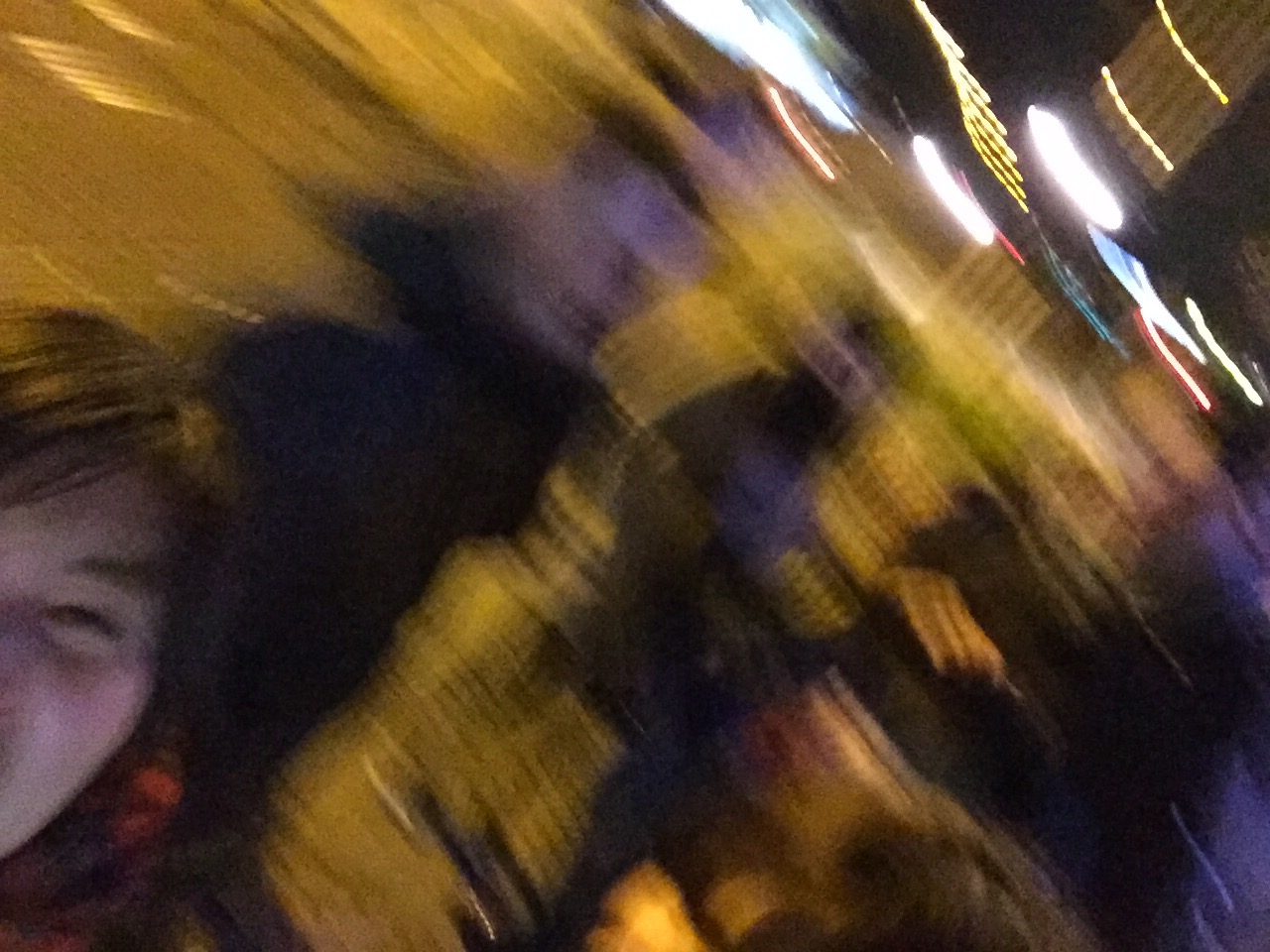The image captures a nighttime outdoor scene, characterized by its overall blurriness and prominent streaks of fluorescent neon lights, indicative of camera or subject movement. On the right edge, there's a partially discernible face of a person with dark black hair and matching eyebrows, possibly of Asian descent. This person is wearing a red and black checkered scarf and a green jacket. The picture appears off-center, requiring a slight head tilt to the right for a clearer perspective. To the viewer's left, a woman with brownish hair and brown eyes is partially visible, adorned in what seems to be a red coat. In the middle, a man can be vaguely identified, but his features are mostly undefined. Beyond these figures, more men are present; one in a black coat and another who seems to be wearing a mask or another scarf. The backdrop includes streaky lights, with some forming vertical lines and others horizontal shapes, suggesting movement. The dark sky reinforces the nighttime setting, and a building with two striped accents on its roof is faintly visible in the top-right corner, completing the scene with a sense of chaotic, blurry vibrance.